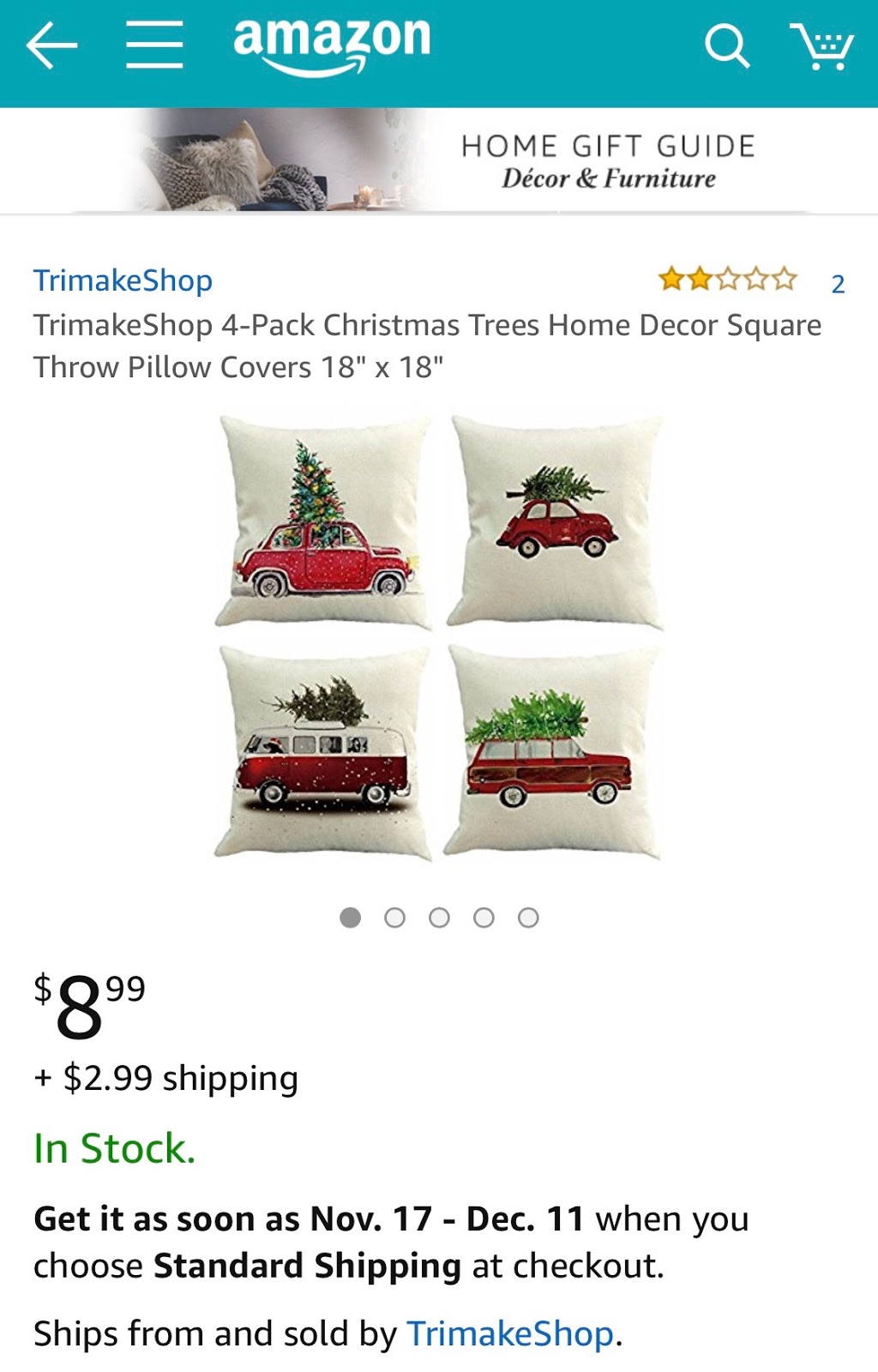Screenshot of an Amazon Mobile App Product Page

At the top of the screenshot, there is a teal blue header. On the far left, a white arrow points to the left, followed by a white hamburger menu. Next to the menu, white text reads "Amazon" with an arcing arrow beneath it. The arrow starts just left of the 'M' and ends with the tip covering part of the 'Z'. On the far right, there is a white magnifying glass icon, followed by a white shopping cart icon.

Below this header is another header with a white background. On the left side of this header, there is a photograph of a grey bed adorned with grey pillows, fading to white on either side. To the right of the photograph, grey, all-caps text reads "HOME GIFT GUIDE." Underneath, in an italicized, non-caps serif font, it says "Decor and Furniture."

A thin grey line separates this header from the product details section, which has a white background. In the top left corner, blue text reads "Trimake Shop." Below this, in grey text, it says "Trimake Shop four pack Christmas trees home decor square throw pillow covers 18 inch by 18 inch." In the top right corner, there are two gold stars followed by three white stars with gold outlines and a blue numeral "2" indicating the product's rating.

Underneath the rating, there is a photograph showing four square pillows arranged in a 2x2 grid. Each pillow has an eggshell white background and features a red vehicle carrying a Christmas tree.